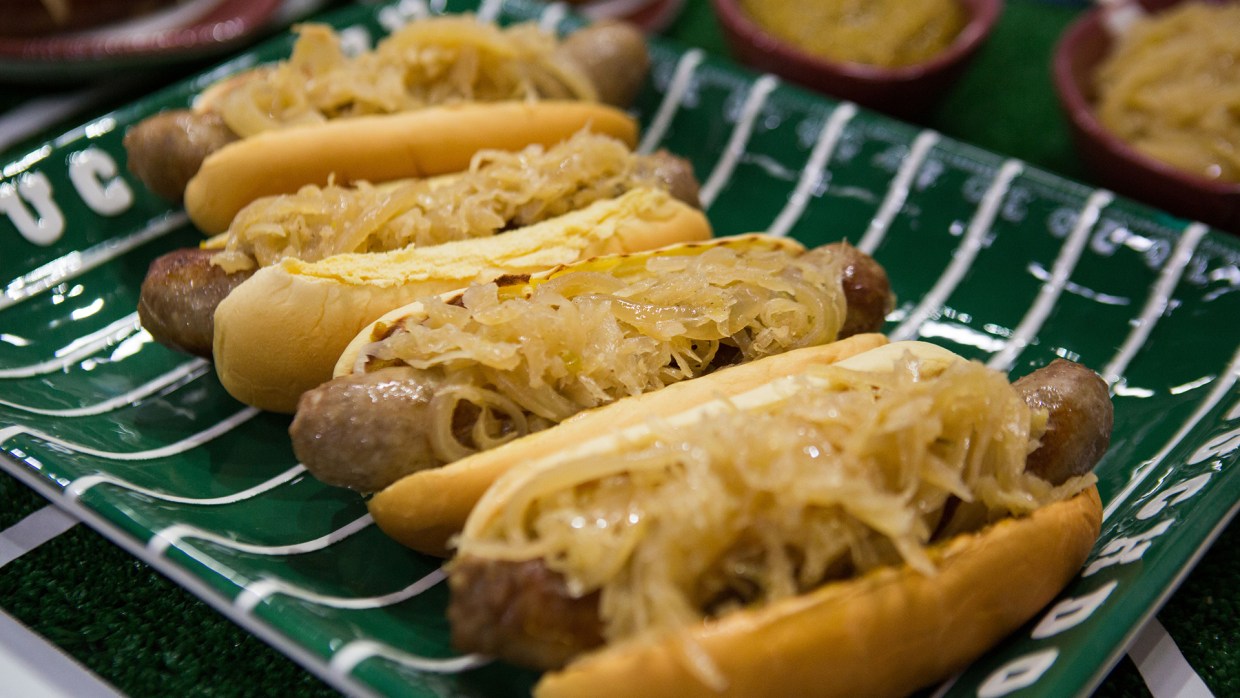The image depicts a green, plastic tray designed to resemble a football field, complete with white yard lines and partially obscured text on either side. On this tray, there are four bratwursts nestled in light brown hot dog buns. The bratwursts are seared, giving them a delicious, browned look, and are topped with glistening, sautéed yellow onions. The tray sits on a tabletop that mimics a football field as well, covered with green, fuzzy material and white tape resembling yard markings. In the blurred background, there are at least two red bowls, possibly filled with more sauerkraut or a yellow dip, enhancing the football-themed presentation.